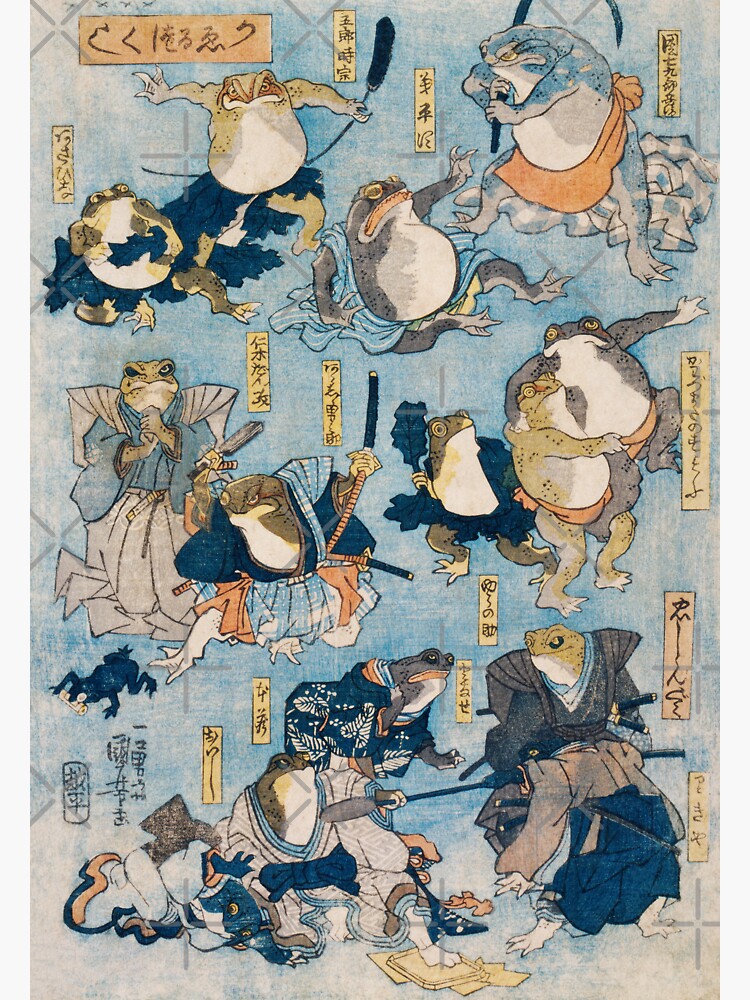In this vibrant, detailed illustration with an aqua blue background, several anthropomorphic toads, dressed in an array of traditional Japanese samurai clothing, are depicted in dynamic martial arts poses. The frogs, with varied skin tones of dark green, gray, and yellow, stand upright on their hind legs, appearing almost human-like. They are clad in colorful robes, including green, pink, blue, white, and dark green with orange accents, some wielding katanas and staffs in their hands. Notably, two frogs in the top left wear green robes, while on the top right, one frog dons a pink robe and another a blue robe. Below these, more toads are seen in combat stances, one wearing a white cloak and another in a dark green and orange cloak, both gripping their katanas. The background is decorated with yellow rectangles featuring Chinese characters, adding to the composition's storied feel. Some frogs engage in sumo-style wrestling or attacking motions, with one frog prominently gripping his sword. The image, reminiscent of an instructional sheet, comic strip, or perhaps a painting from the 1970s, is further embellished with Japanese or Chinese text, providing an additional layer of cultural depth.